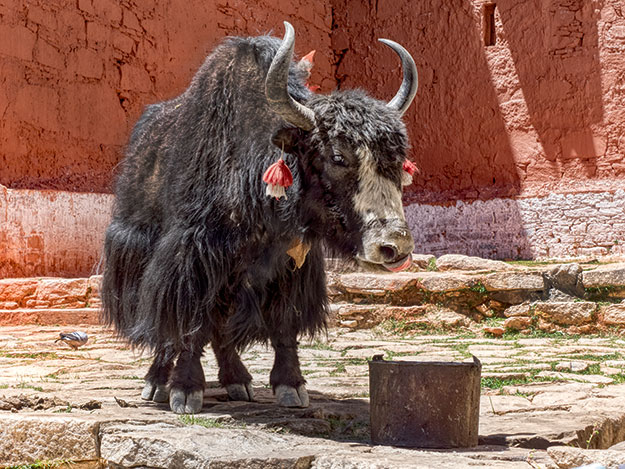In this vibrant image, the central focus is a large, shaggy animal resembling a yak with distinctive features that could also suggest a muskox. This creature, with its gray, long hair and prominent hump, stands out against a backdrop of rustic, reddish-brown adobe-like walls. The animal's horns are long and curve upwards, and its ears sport unusual red and white earring-like tags that resemble mushrooms or umbrellas. Its expressive face, with a white streak down its nose, appears to be leaning over a stone dish or water container. The scene is set on a stone or brick path with scattered rocks and patches of grass, indicating an outdoor environment. A small bird is visible on the ground to the left, adding an extra layer of detail to the scene, hinting at a serene, possibly zoo-like setting under sunny skies.